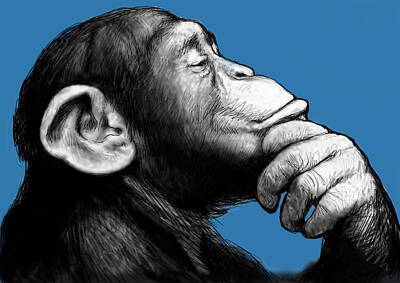The image is a black and white drawing of a chimpanzee set against a bright blue background. The artwork portrays a pensive chimpanzee in a profile view, looking to the right. The chimpanzee's large ears are prominent and uncovered by his long black hair, while his grayish face, hands, and ears stand out against the blue backdrop. Notably, the area around his nostrils, mouth, and his raised left hand, which supports his chin in a thoughtful pose, lack hair. His eyes are closed, reinforcing the contemplative mood, reminiscent of the famous "Thinking Man" statue. The striking use of blue highlights the introspective nature of this pop art drawing.